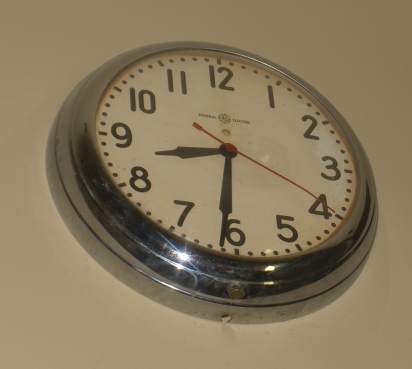This image showcases an aged analog wall clock with a distinctive nostalgic charm. The clock, likely wearing the marks of time, displays a slightly rusty and spotty face, indicative of its age. The clock's frame is silver, bordered with a typical chrome finish, adding a touch of vintage elegance. Its white face is accented by a red second hand, juxtaposed against the stark black hour and minute hands. The clock features plain, easily readable numbers, ranging from 1 to 12. The time shown is 8:31. At the center of the clock face, there is an emblem resembling a 'G' in cursive, flanked by the words "General Electric," highlighting the clock’s heritage brand.